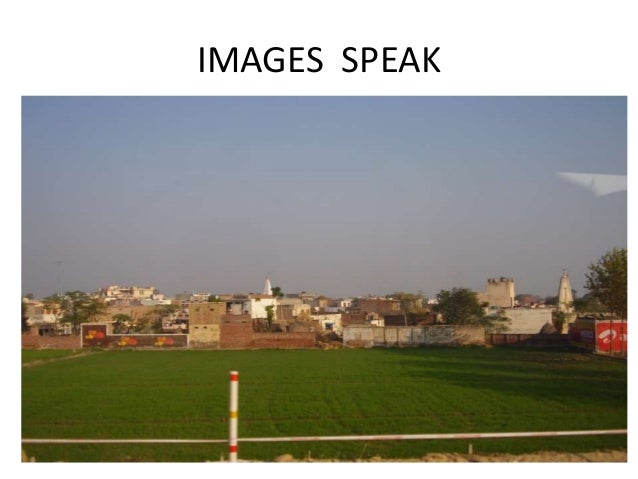The image depicts a wide, green sports field, possibly a practice or recreational area, with recently mowed short grass. The field is bordered in the foreground by a low white fence bearing reflective red and yellow tape. Two faint horizontal lines on the grass suggest tire tracks. In the background, a small town or village is visible, displaying a variety of older, indistinct buildings, including industrial-looking structures and houses perched on a hill. Notably, there is a central piece of architecture, a small white obelisk with a yellow or orange top. Additionally, a trailer is parked on the right side of the image. Above the scene, the sky transitions from a hazy blue to a darker hue, indicating either early morning or late evening. The words "images speak" are inscribed in thin black writing at the top. The entire image is suffused with a calm, almost nostalgic atmosphere, highlighting both human-made and natural elements in a seamless blend.